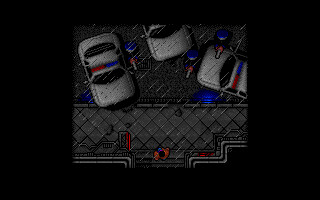This image depicts a scene from an 8-bit video game, viewed from a top-down perspective. The central character, who sports an orange shirt and a baseball cap, is seen standing on a sidewalk. Surrounding him are three police officers with their firearms drawn, aiming directly at the character. Next to the sidewalk, three police cars are parked in a line. The scene is devoid of any additional text or score, focusing entirely on the intense standoff. The simplistic pixelated style and the vibrant colors are characteristic of classic 8-bit video games, evoking a sense of nostalgia for early gaming aesthetics.